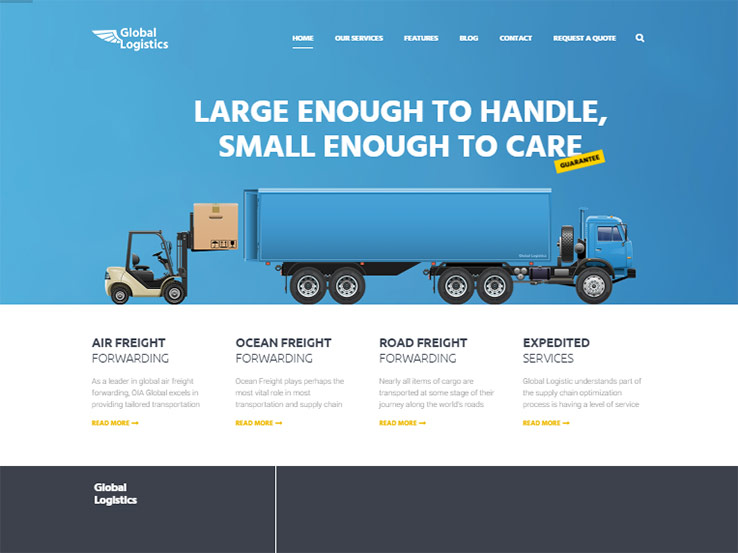The image features a detailed layout divided into two main sections. The top half has a blue background with white text on the upper left corner that reads "Global Logistics". Adjacent to this text is a white logo shaped like a wing. Across the top are navigation buttons labeled "Home", "Our Services", "Features", "Blog", "Contact", "Request a quote", and a search icon.

Prominently displayed in the center, the slogan "Large enough to handle, Small enough to care" stands out, with the word "Guarantee" highlighted in black against a yellow background. Below the text is an image of a blue truck facing right. A yellow forklift on the left side is seen loading a brown box into the back of the truck.

The bottom half of the image has a white background with several subtopics, each marked with a yellow bullet point. They are:
1. **Air Freight Forwarding**: Describes CMA Global as a leader in Global Air Freight Forwarding, excelling in providing tailored transportation.
2. **Ocean Freight Forwarding**: Highlights the critical importance of ocean freight in transportation and the supply chain.
3. **Road Freight Forwarding**: Notes that nearly all cargo is transported along roads at some stage during its journey.
4. **Expedited Service**: Mentions that Global Logistics understands the necessity of having optimized supply chain services.

At the bottom left corner, there is a black rectangle featuring the text "Global Orange" in white.